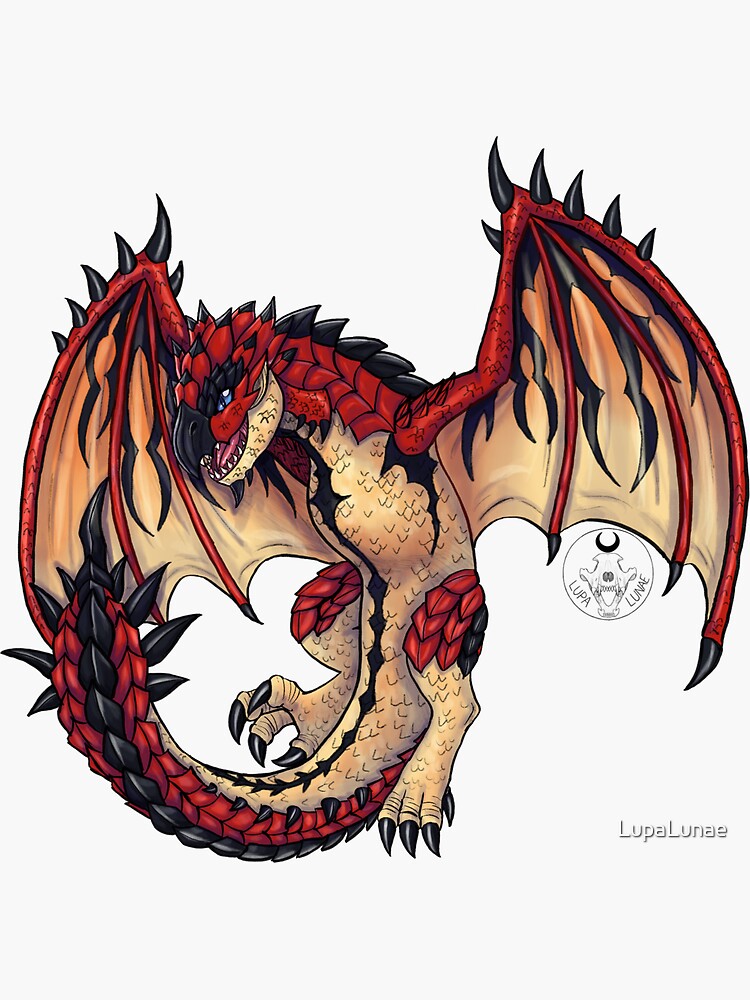The image depicts a detailed cartoon drawing of a dragon centered on a white background. The dragon stands on clawed feet, one foot raised, and the feet are beige with large black claws. The dragon has red scales with black and red details on its wings, and red highlights on its knees. A black line adorned with diamond shapes runs from under its chin down the length of its belly to its tail. The dragon’s head features a prominent black beak, and it sports sharp white teeth with small molars. Its eyes are black with blue irises. The creature's wings are outstretched, displaying a mix of black and red lines, giving an impression of flight or posing. Additional black spikes can be seen along its neck, back, and tail, and white accents are visible beneath its wings. Text beneath the image reads "Lupa Lunae," and there is an additional circular detail near the dragon's back. This dragon exudes the dynamic flair typical of characters from video games.